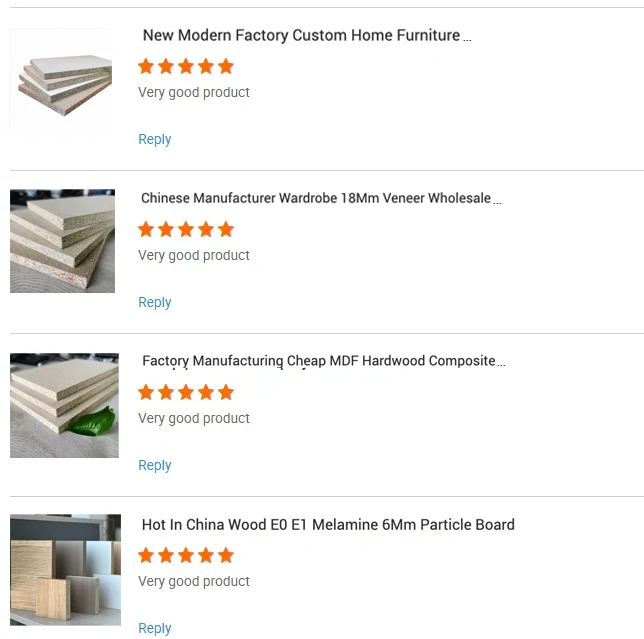Here is a revised and detailed caption for the image described:

------

The photo showcases a collection of four items. At the top, there is an image of a sleek, modern piece of factory-made home furniture. Highlighted in bold, black font, it boasts a five-star rating and a glowing review stating, "Very good product." To the left of this item is an image depicting a pile of raw wood.

The second item features a well-crafted Chinese-manufactured wardrobe with an 18 mm veneer, available at wholesale prices. Accompanying this, like the first, is an image of a pile of wood. This product also carries a five-star rating and is praised as a "Very good product."

Moving further down, the third item appears to be three finished pieces of wood – akin to those found in a build-it-yourself furniture kit. This piece is identified as factory-manufactured cheap MDF hardware composite and is similarly awarded five stars for its quality.

Finally, the last item presents itself as a hot commodity in China – a wood panel with EOE1 melamine, made from 6 mm particle board. Like the preceding items, this product ensures high quality.

Each product in the photo is backed by a consistent five-star rating, underscoring their exceptional quality and desirability.